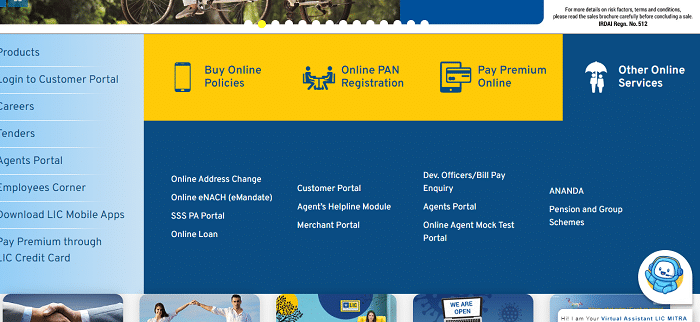A detailed screen capture image illustrating various elements related to an online insurance portal. 

At the top part of the image, there is a partial view of a person’s foot on bicycle pedals along with a glimpse of the bicycle wheels. Below this, there is a row featuring several white circles and a solitary gold circle. Off to the side of this section, a blue bar is present. In black font, it is written: “For more details on the risk factors,” but the remaining text is blurry and unreadable.

Further down, a gold box contains navy blue font reading “Buy Online Policies,” and there is an icon of a cell phone. Next is the text “Online PM Registration.” Nearby, there is an icon depicting two people talking at a table, accompanied by the text “Pay Premium Online” with a small graphic combining a cell phone and a credit card.

There’s also a blue box with white font announcing “Other Online Services," with an image of two people under an umbrella beside it. Following this, a series of white submenu options are listed: "Online Address Change," "Online ENACH," "E-Mandate," "SSS," "PA Portal," "Online Loan," "Customer Portal," "Agent’s Helpline Module," "Merchant Portal," "Developers," "Officers," "Bill Pay," "Inquiry," "Agent’s Portal," "Online Agent Mock Test Portal," "Ananda," "Pension and Group Schemes." Additionally, a friendly-looking blue robot icon with a headset and a white face is visible.

At the bottom of the screen, there’s a series of images: a blue airplane, a box displaying “We Are Open” on a laptop screen with blue virus particles in the background, a gold and blue box with an image of a woman, a man and a woman holding hands dressed in white, and two people in suits shaking hands.

Above this section is another menu with various submenus written in blue font on a white background, which includes options like "Products," "Login to Customer Portal," "Careers," "Lenders" (assumed), "Agent’s Portal," "Employee’s Corner," "Download LIC Mobile Apps," and "Pay Premium through J<CreditCardName>."

This image provides a comprehensive view of an online insurance portal with various features and options displayed in a clear, organized manner.